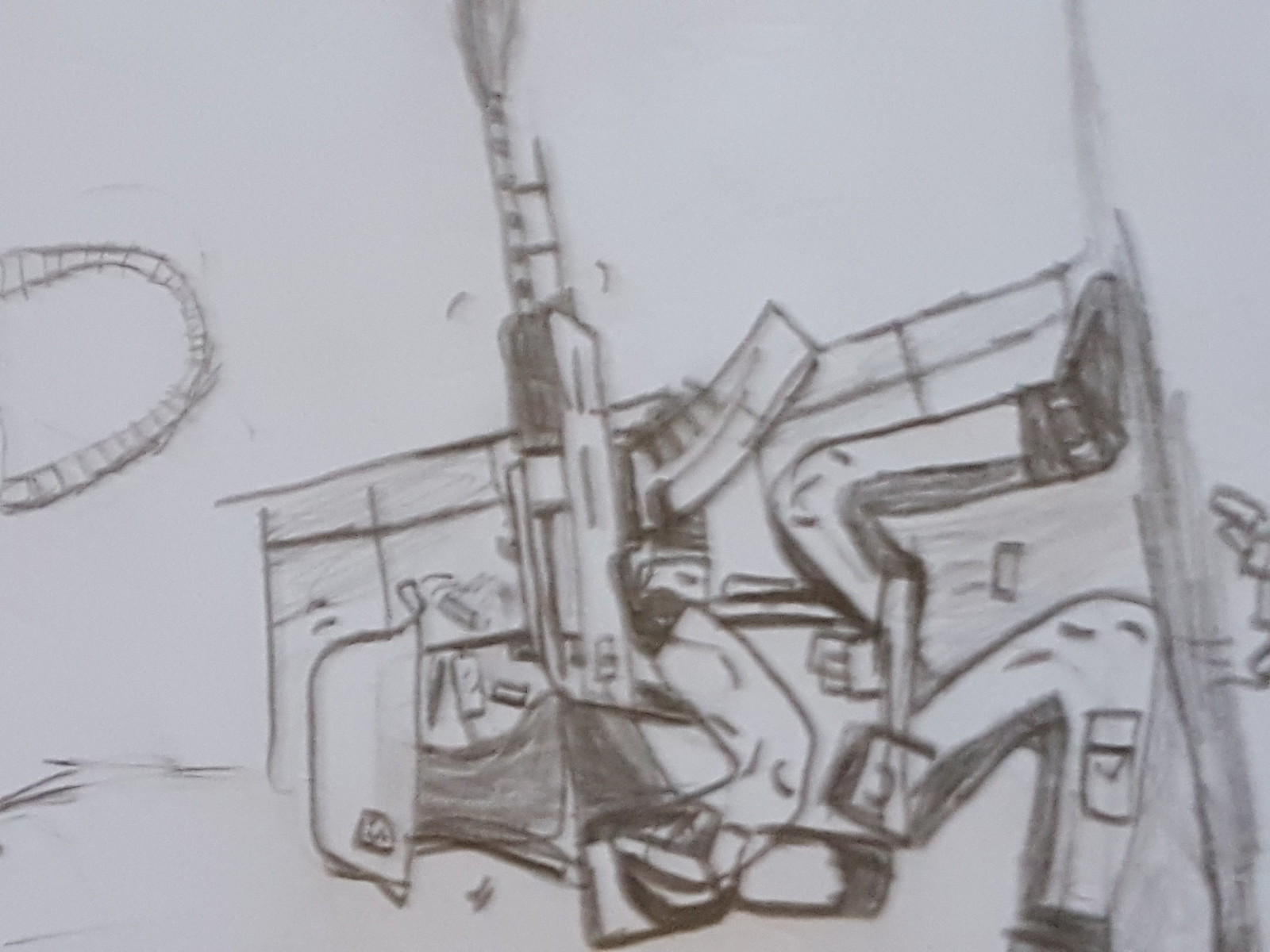This is a highly detailed pencil drawing on paper depicting a soldier in an active combat scenario. The soldier, identifiable by their helmet and tactical goggles, has shoulder-length hair and is clad in a military uniform complete with cargo pants and rugged boots. Positioned behind a protective wall, the soldier is captured in a dynamic kneeling stance—one knee on the ground and the other raised—as they fire an automatic weapon. The intense moment is further emphasized by the small, yet significant detail of a spent ammunition cartridge in mid-air above the soldier's head. Despite the image being oriented sideways, the intricate details remain discernible, showcasing the artist's meticulous attention to realism and movement.